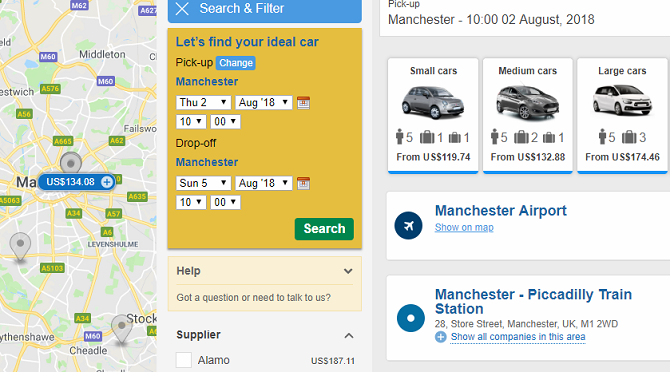This image is a detailed screenshot from a car rental agency's online booking platform. On the far left, there's a column displaying a map with various cities listed. Prominently, at the center of this map, a blue oval indicates a price, labeled "U.S. Dollars 134." 

The column next to it features a blue header titled "Search and Filter." Underneath, the text "Let's find your ideal car" is inviting users to make selections. It then shows "Pick up" with a blue button labeled "Change" next to "Manchester," set for Thursday, August 2nd at 10:00 AM. The "Drop off" details note Manchester again, on Sunday, August 5th at 10:00 AM. At the bottom of this section, a green "Search" button is prominently featured within a gold rectangle. 

Adjacent to this is a pale yellow "Help" rectangle with a dropdown menu that invites users to ask questions or contact support. Below this, there’s a subheading "Supplier: Alamo," and directly opposite it, the cost "U.S. Dollars 187.11" is displayed.

The third column details the available cars for pick-up in Manchester, showcasing three images of cars classified by size: a small car starting from $119.74, a medium car from $132.88, and a large car from $174.46. Below this, the white triangle section mentions "Manchester Airport" with an option to "Show on Map." Further down, it lists "Manchester Piccadilly Train Station" with the address "28th Street, Manchester, UK, M12WD." Finally, at the very bottom, there’s a button for "Show all companies in this area."